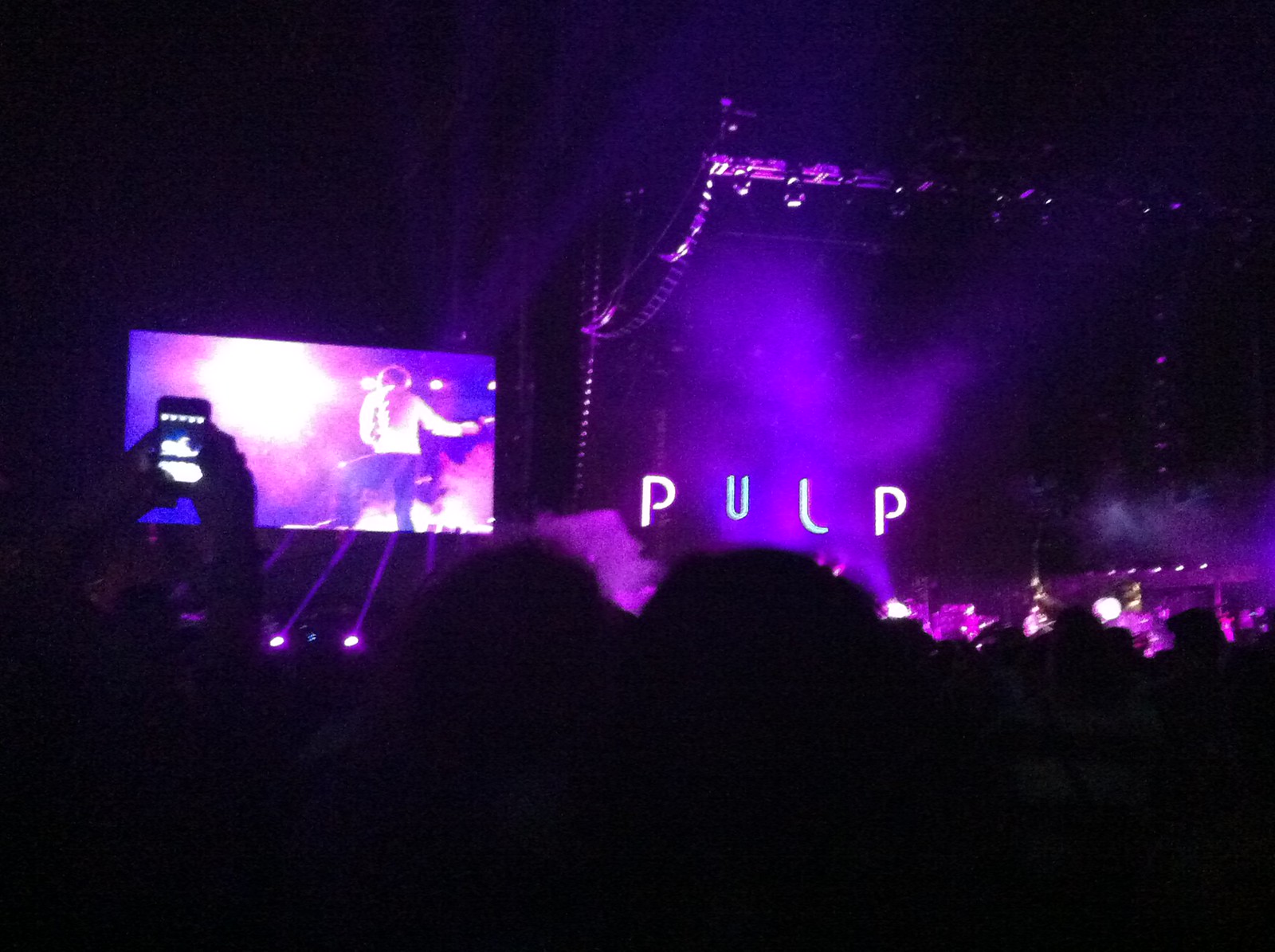The image captures a concert scene bathed in deep purples and shrouded in darkness. The dense, pitch-black crowd stretches into the foreground, punctuated by the faint outlines of heads and a silhouette of a man holding up a smartphone to record the spectacle. At the center stage, roughly 50 feet away, vibrant purple lights beam through a haze of smoke, giving it a surreal purple tint. Illuminated in brilliant purple letters at the heart of the stage is the word "PULP." Further left, a large screen projects the image of a performer dressed in a white shirt and black pants. The performer's back is to the audience, obscured by the intense purple glow, making his specific features indistinguishable. Above the stage, beams of light crisscross through the air, stemming from spotlights on the ground, casting dramatic shapes through the smoky atmosphere. The concert space is dark save for the dazzling, almost celestial, purple illumination that engulfs the scene, transforming it into a vivid, dreamlike spectacle.